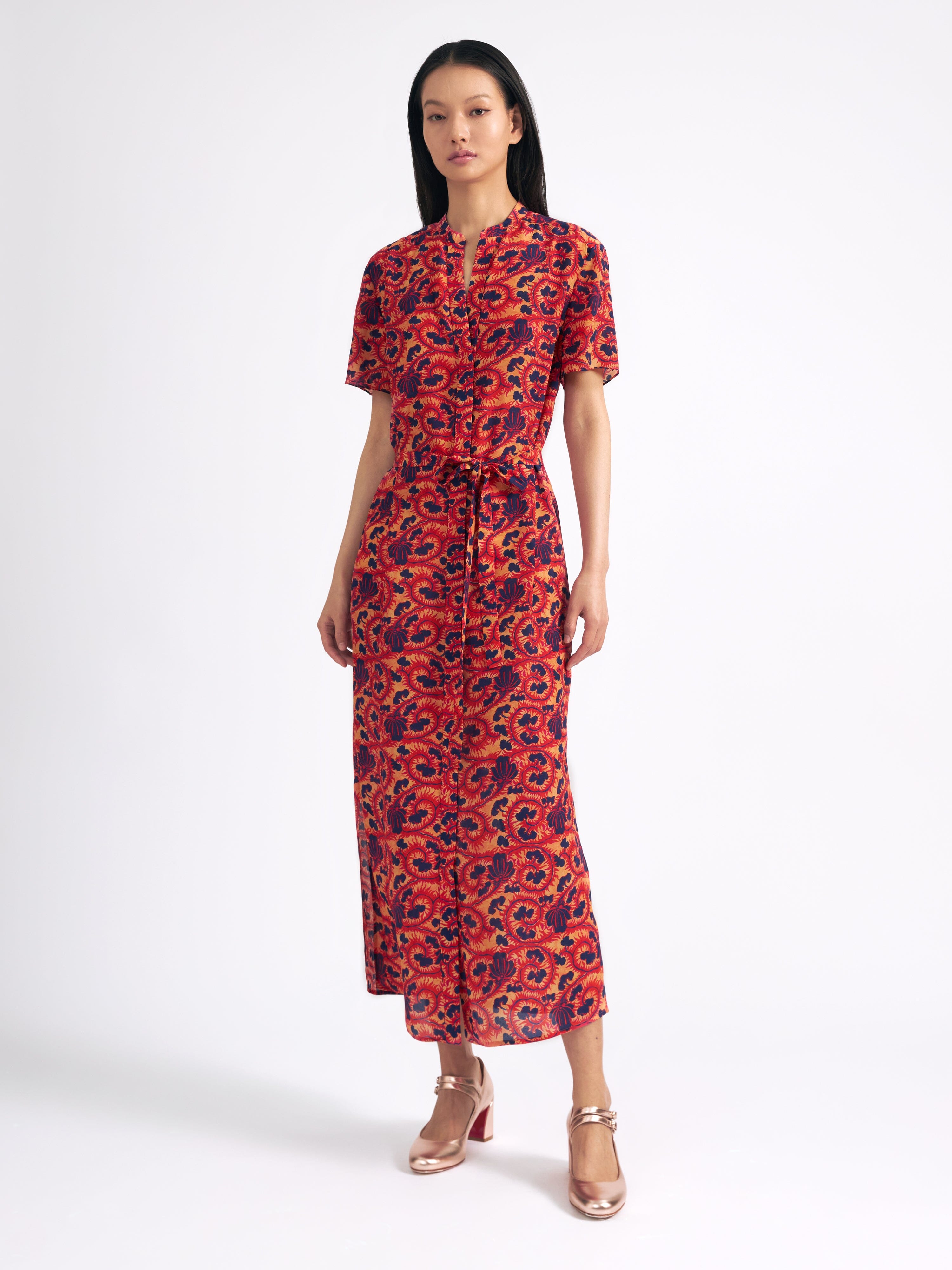This is a portrait mode photograph of a statuesque, tall Asian woman standing against a light gray background. She has long, black hair that flows behind her neck and wears pink lipstick. Her dress is a striking multicolored floral ensemble featuring shades of orange, red, and deep purple. The dress, which appears to be made of cotton, extends almost to her ankles and has a vibrant, intricate pattern with swirling shapes, reminiscent of Paisley. It is short-sleeved, with sleeves ending just above her elbows, and buttons up near the top, exposing a small part of her chest near the clavicle. A ribbon tied at her waist cinches the dress, giving it a wrap-around appearance. She is wearing elegant, shimmery shoes that appear to be a blend of silver, gold, and rose gold, with straps across her ankles and thick heels. The woman stands alone, precisely centered in the image, with her shadow extending out towards the left at the bottom near her shoes. Her arms hang straight down past her waist, emphasizing her poised and composed presence.